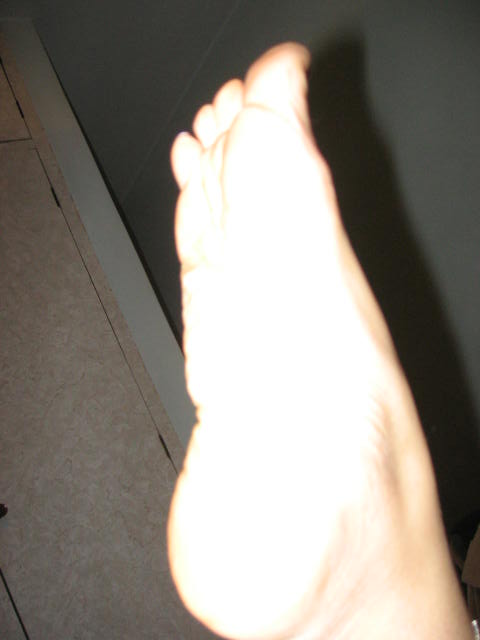This tall, rectangular photograph offers a close-up view of a foot, bathed in a bright flash that obscures finer details. Positioned slightly to the right within the frame, the foot displays light skin and hints of an ankle in the bottom right corner. The heel anchors the foot at the bottom, with the toes spread out towards the top. Although the big toe, facing the camera, and three additional toes are visible, the fourth toe remains out of sight. The background reveals a floor of light beige tilting diagonally to the top left, adjacent to what's possibly a greenish-gray or tan wall. Notably, a stark black shadow of the foot is cast against this wall, hinting at depth and providing contrast. There is also an impression of a structure, potentially a closet, with visible hinges and a white border, leading to what seems to be a dark hallway.